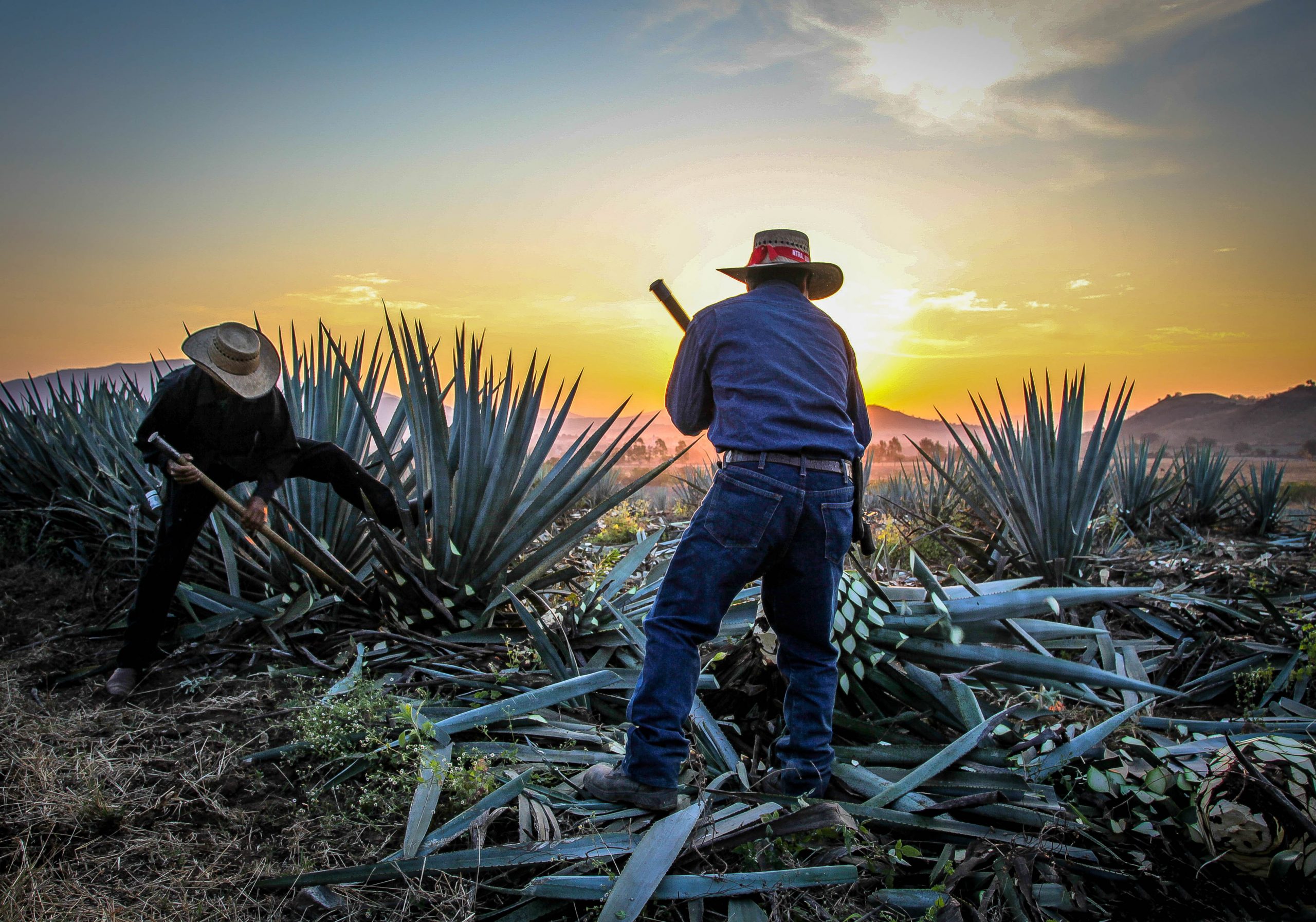In a vibrant sunset setting in the desert, two men, likely migrant workers, are diligently harvesting yucca or agave plants. The sky transitions from blue to stunning bands of orange, pink, and yellow as the sun dips behind distant mountains. Both men are dressed in denim; the man in the foreground dons blue jeans and a denim shirt, while the other is in black jeans. Both wear work boots and straw hats, with the man in the center distinguished by a red bandana wrapped around his hat. The man in the foreground has already sheared a large yucca plant, scattering its green leaves across the dry, grass-covered ground, while the man to his left focuses on dislodging another plant from the soil. Behind them, the landscape is dotted with trees and takes on a brownish hue, adding to the rustic charm of the scene.